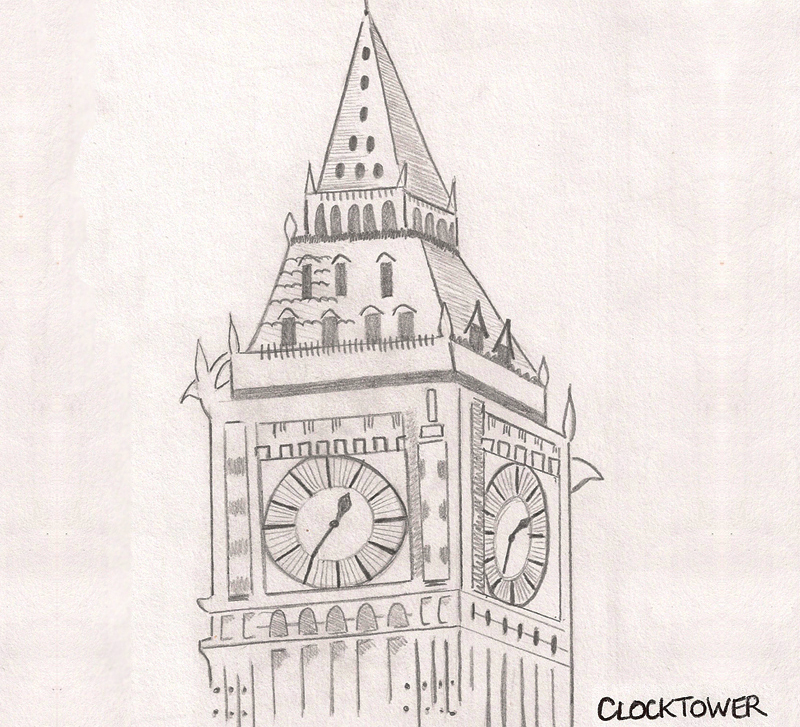This is a detailed, color pencil drawing on high-quality textured paper, depicting the top portion of the Elizabethan Tower in London, particularly focusing on the Big Ben clock. The drawing captures the section of the tower from just below the two visible clock faces to the pinnacle of its triangular, steeple-like roof. Each clock face shows a different time, and the intricate detailing includes multiple dormer windows below the steeple, some of which feature small balconies. The tower is illustrated as a square, extruded structure with minimal shading, emphasizing the stone-like texture of the building. Notably, the bottom right corner of the drawing is labeled "clock tower."